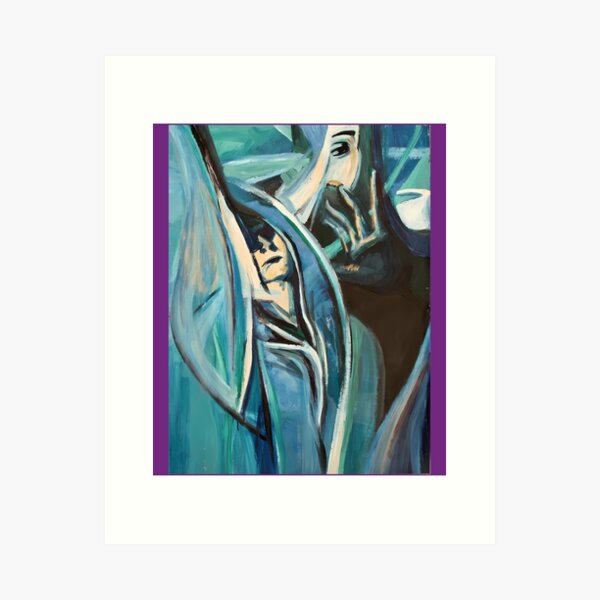This is a collared photograph of a painting matted in a white frame, set against a white background. The painting, predominantly in blue, turquoise, and green hues, features two thick purple vertical stripes along the left and right borders. In the center, the abstract artwork reveals two figures. One figure, obscured partially by heavy green-blue brushstrokes suggesting leaves or some other organic forms, shows a white face where only the nose and mouth are distinctly visible. The eyes are uncertainly covered by either hair or abstract lines. In the upper right-hand corner, a second figure appears, characterized by a large hand with partially visible black glove and fingerless tips, half-veiling her face as if pushing away or shielding herself. The composition suggests dynamic tension, with intricate vertical lines and curves blending these elements into an evocative, emotive tableau.